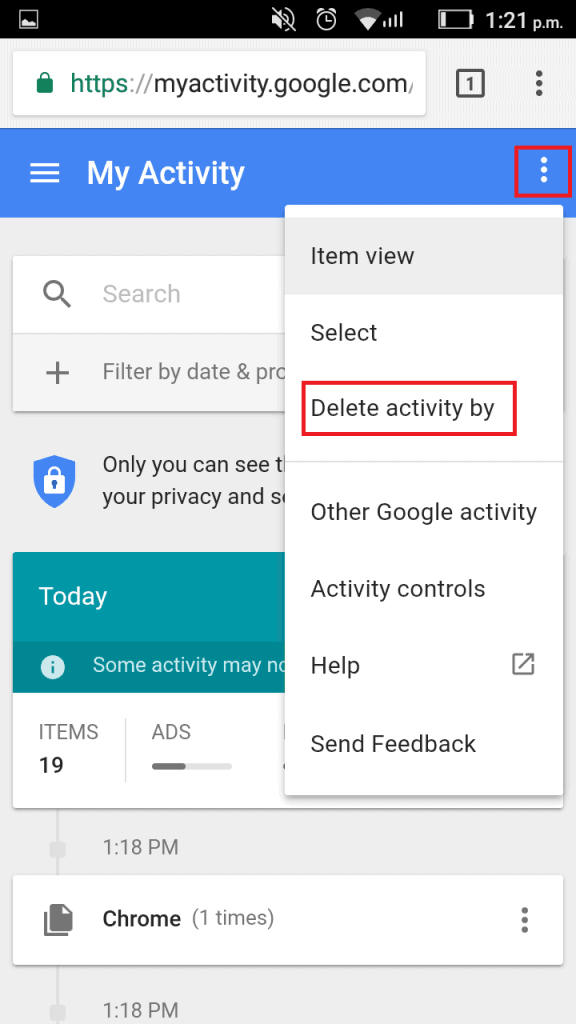This image is a screenshot taken from someone's cell phone, displaying the "My Activity" page on the Google Activity website (https://myactivity.google.com). 

At the top of the screen, there is a black status bar featuring various icons. Starting from the left, there is an icon resembling a picture. Moving towards the middle, there are icons indicating that the sound is off, the current time is 1:21 p.m., the network signals (Wi-Fi and bars), and the battery level, which appears to be very low.

Below the status bar, the "My Activity" section is highlighted within a royal blue rectangle. On the far right of this section, there are three vertically aligned white dots representing a menu. This menu has been activated and a red rectangle has been drawn around it.

The active menu displays a dropdown box that includes the following options: "Item view," "Select," "Delete activity by," "Other Google activity," "Activity controls," "Help," and "Send feedback." The "Delete activity by" option is also encased within its own red rectangle, emphasizing it as the selected choice.

Further down, a teal section labelled "Today" is partially visible, with the text indicating some activity may not be fully shown, although it is cut off at this point.